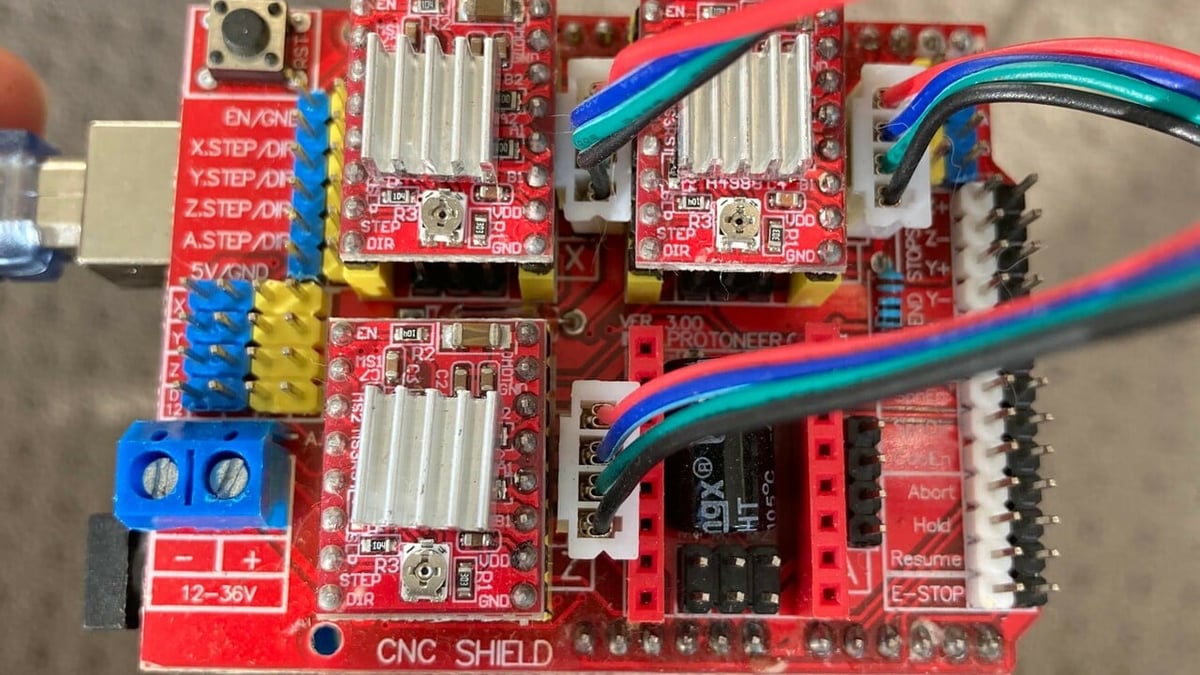This full-color, close-up photograph, taken indoors with artificial lighting, features a horizontally rectangular image with no border and a matte gray background that is out of focus with holes. The focal point is a red CNC shield circuit board, densely packed with white text and various components. Among the labeled areas, it includes marking such as "X step," "Y step," "Z step," "A step," "12-36V," "e-stop," "resume," "hold," and "abort." The circuit board has white connectors that house a multitude of colorful wires—red, blue, green, and black, including a blue wire with a white stripe. These wires connect to three distinct sections of the board. In the upper left-hand corner, only the tip of a person's finger is visible, pushing a blue fuse into the gray portion of the board. A USB-C connection is present on the left side, and a switch is located at the top left, indicating possible use for a small computer or robotic application.